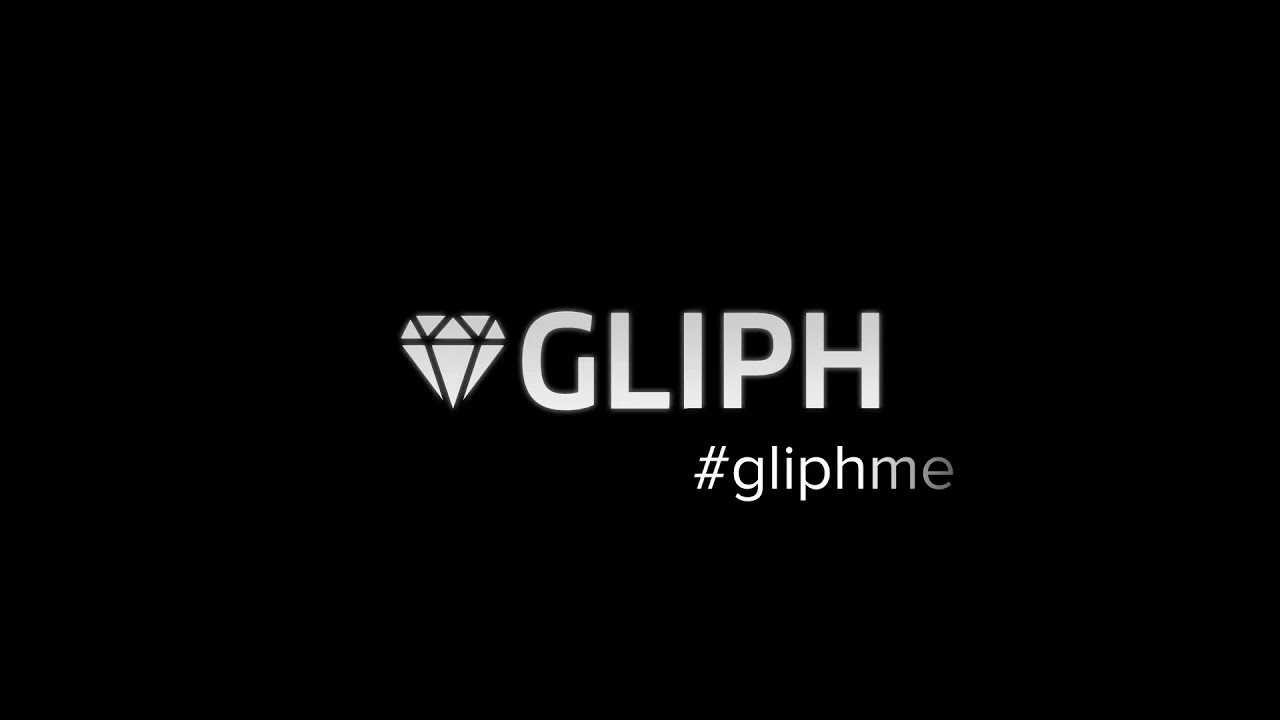The image features a minimalist, predominantly black background with a centrally placed graphic design. In the middle, there is a diamond icon composed of multiple interconnected triangles. This icon is positioned to the left of the bold, uppercase text "GLIPH" in a near-white, silver-gray color. Below this text and offset to the right, starting beneath the "I" and extending towards the "P," is the hashtag "#glyphme" in lowercase. The entire scene is encased within a horizontal rectangular shape, emphasizing its stark and simple design.